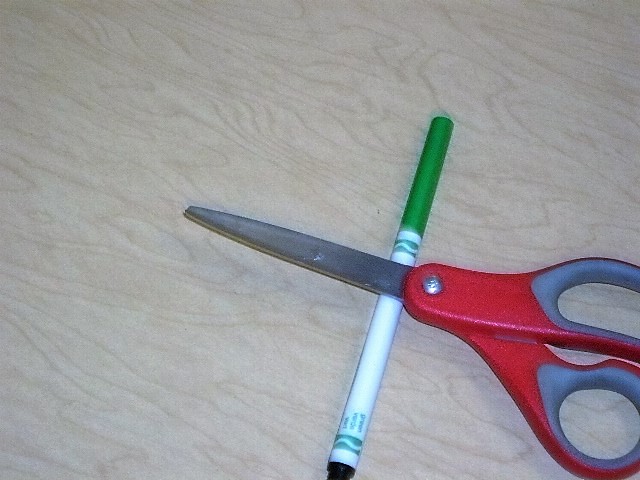This photograph captures a simple scene featuring a pair of child safety scissors and a Crayola marker laying on a light-colored wooden table, with visible wood grain patterns. The background is uniformly the table surface, giving the image an uncomplicated and clear backdrop. Positioned from the bottom right, the red-handled scissors with gray cushion grips are shown closed and pointing diagonally to the upper left. Their metal blades rest over the green marker, which lies vertically with its green cap pointing upward. The marker is white with green bands typical of a Crayola design. The image is somewhat dimly lit and not the sharpest in focus, but it effectively showcases the two objects against the light woodgrain background.